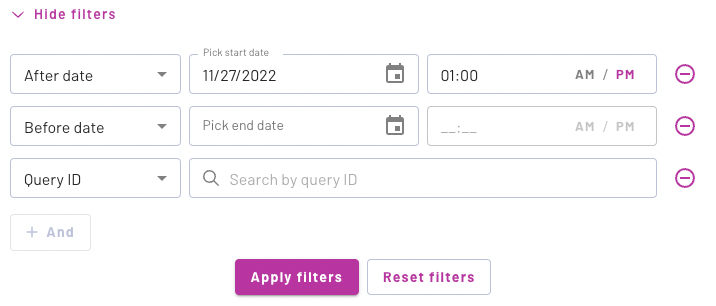The image depicts a horizontally elongated interface with multiple filter options for querying data. 

At the top of the image, there is a purple button labeled "Hide Filters." Below it, a drop-down menu can be accessed. 

The first filter row begins with a label "After Date," accompanied by a prompt to "Pick Start Date." The field is populated with the date "11/27/2022" and is flanked by a calendar icon. Adjacent to this, the time is set to "1 PM," highlighted in purple.

The second filter row is labeled "Before Date" with a prompt to "Pick End Date." This row includes a calendar drop-down; however, no date or time is selected.

In the third row, there is a filter field labeled "Query ID," which suggests users "Search by query ID" in placeholder text, displayed in gray. This field is currently empty.

Each of these rows features a purple circle with a line through it at the end, possibly indicating an option to remove the specific filter.

At the bottom left of the interface, there is a "Plus Add" button featuring a white background and gray lettering. 

Finally, there are two main action buttons at the bottom of the interface: one purple button with white lettering that says "Apply Filters," and a white button with purple lettering outlined in gray that reads "Reset Filters."

The overall background is white, creating a clear contrast with the almost black or gray font used in the fields, while purple highlights emphasize specific interactive elements.